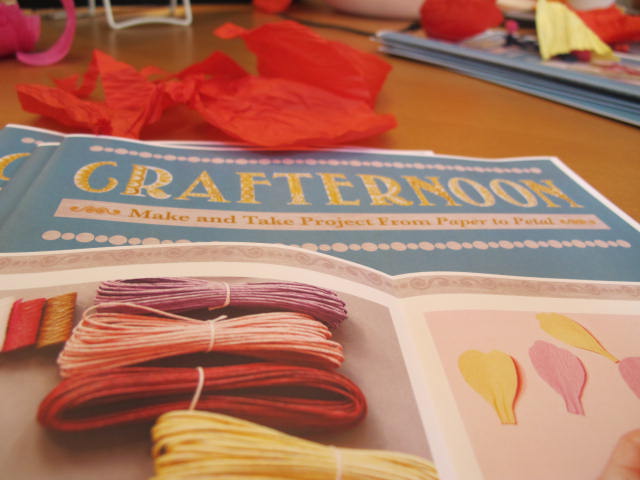This photograph captures a charming craft scene, featuring a blue book titled "Crafternoon" prominently positioned in the background. The book’s cover is emblazoned with vibrant yellow lettering. Below the title, in a white box with matching yellow text, are the words "Make and Take Project from Paper to Petal." Resting on top of the closed book is an open craft book, displaying an engaging project. The left page showcases an array of colorful threads—purple, pink, red, and yellow—while the right page exhibits cut-out shapes of flower petals, ready for assembly.

The setting includes a rustic wooden surface, possibly a table, adding warmth to the scene. In the top left corner, crumpled and then neatly opened red tissue paper adds a touch of vivid texture. Nearby, another stack of similar blue books or magazines sits, contributing to the creative ambiance. The top right of the image reveals additional stacks of books or magazines, adorned with more yellow and red tissue paper, suggesting ongoing or upcoming crafting activities. The overall composition invites viewers into a cozy, imaginative crafting environment.